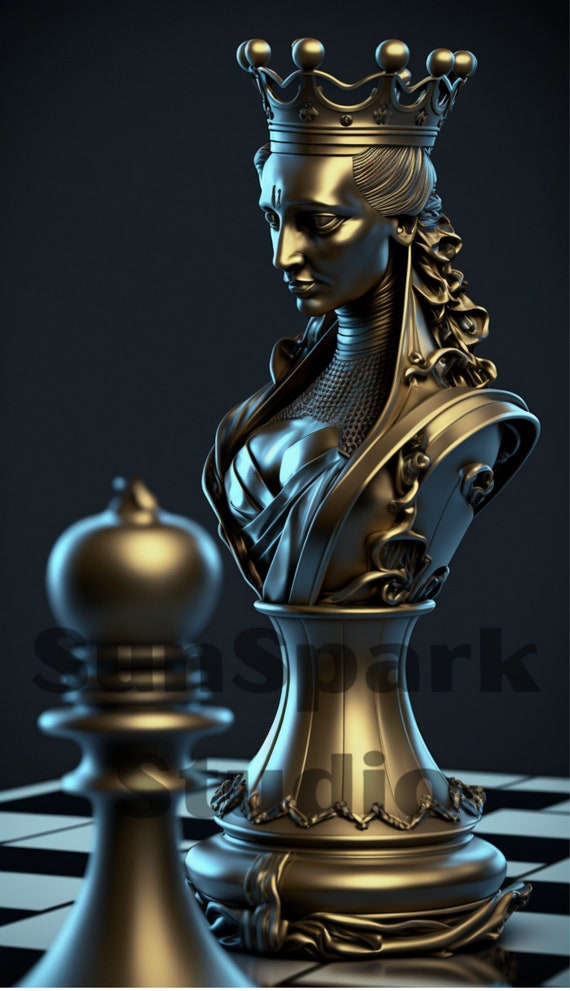The image features a prominent and intricately detailed queen chess piece set against a black background. The queen, situated centrally in the frame, faces toward the left. Her visage is adorned with a regal crown and cascading long hair, reminiscent of the finely detailed queens depicted on a deck of cards. This chess piece, shining with a brassy or die-cast metallic luster, extends from the top of her crown down to her chest area, emphasizing its imposing stature that fills the frame vertically. Below, at the base of the image, lies a black and white checkerboard pattern. Additionally, in the lower left foreground, there is another smaller chess piece, likely a pawn or bishop, contributing to the overall composition. In the center of the picture, the text "Sun Spark Studio" is displayed, adding an identifying mark to the artwork. The sophisticated design and shimmering metallic finish of the pieces suggest a high level of craftsmanship, possibly indicating that the chess pieces are part of an elaborate and visually striking set.